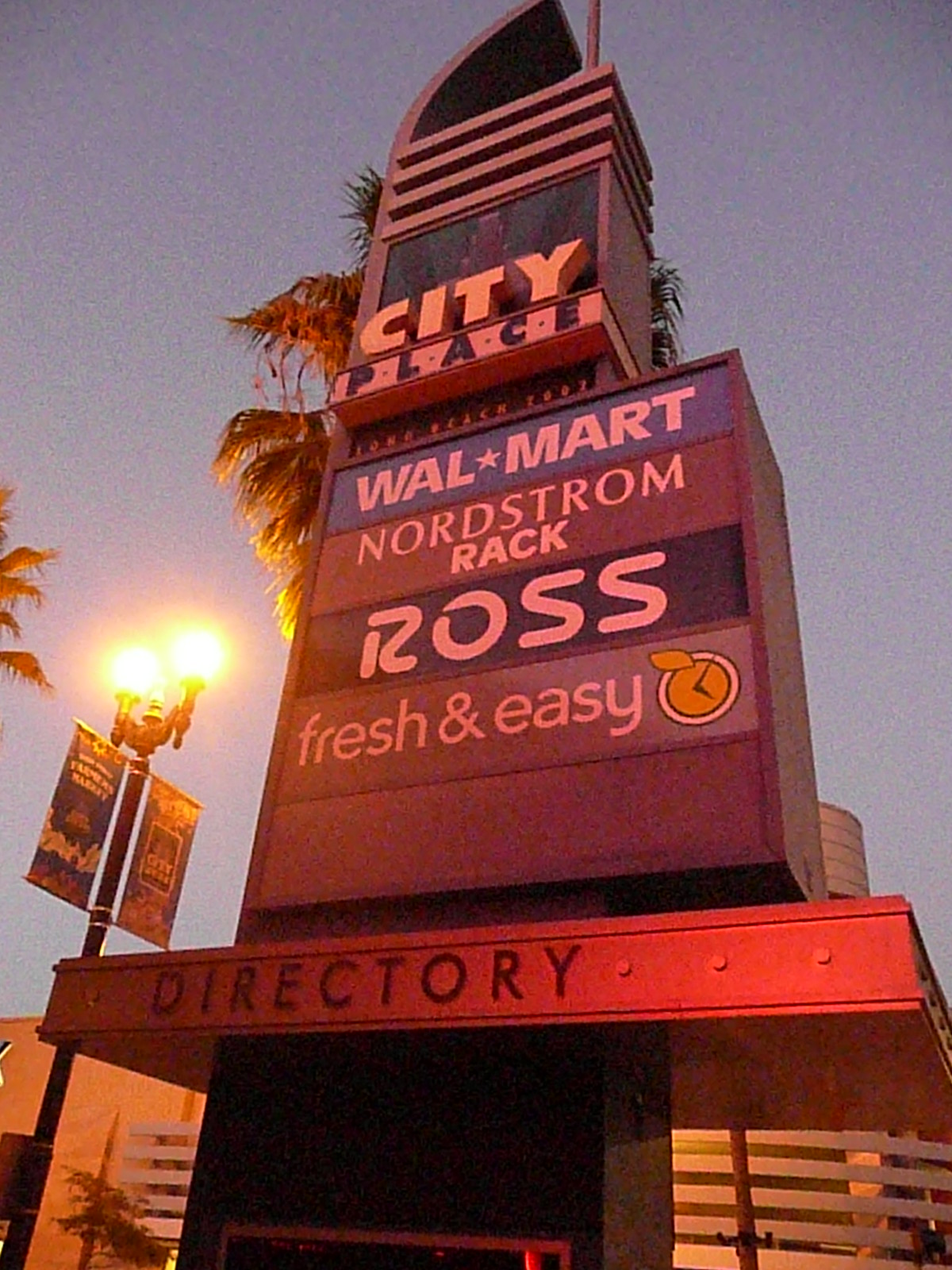The image features a backdrop that blends grey and blue hues, reminiscent of a cloudy sky. Dominating the left side of the frame is a tall pole adorned with two banners. Attached to the pole is a light fixture that extends horizontally at the top, illuminating both left and right directions.

At the center bottom of the image, the text "Directory" is visible, accompanied by a series of dots. Flanking this text on both sides are metallic accents in shades of orange and silver.

An eye-catching clock branded "Fresh and Easy" sits prominently in the background, serving as a focal point. Above this clock are multiple large white texts in succession: "Ross," "Nordstrom Rack," "Wall Star Mart," and at the very top, "City Place." To complete the scene, several palm trees are visible, adding a touch of nature to the urban setting.